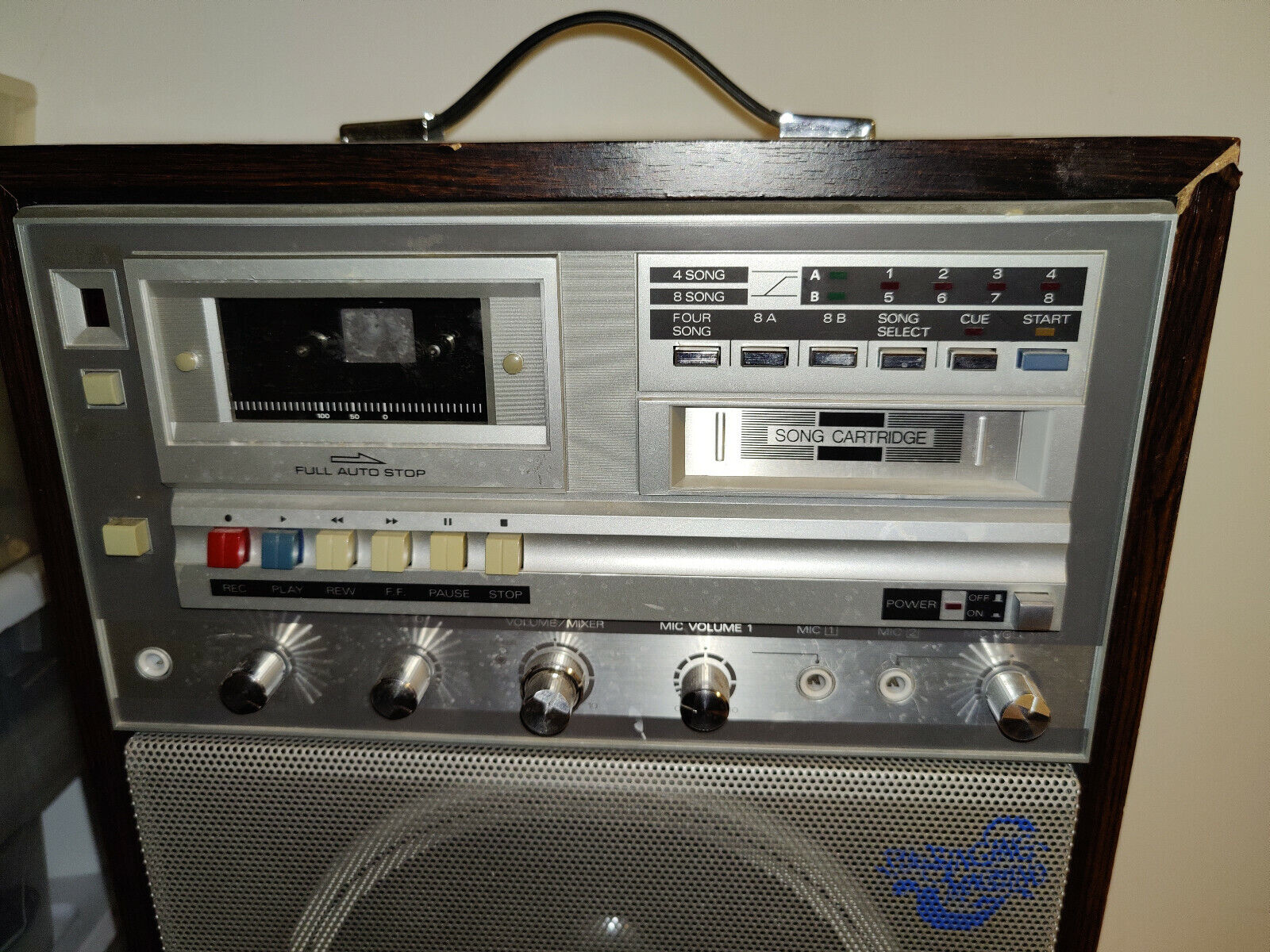This image showcases an old, vintage stereo system integrated with an 8-track player and radio, set against a light brown wall. The stereo features a handle on top, suggesting portability. The device's front interface is framed with a silver border and includes a myriad of buttons and knobs. Prominently displayed is a rectangular section labeled "Song Cartridge," accompanied by controls for "4 Song," "8 Song," "A and B," and a numbered selection from "1 through 8." Additional buttons include "Song Select," "Cue," and "Start." The upper left section houses a closed cassette player marked "Full Auto Stop," with a black screen and white vertical dashes. Below this are various colored buttons for "Stop," "Play," "Forward," "Reverse," and "Pause," along with multiple silver knobs, likely for volume and microphone input adjustments. The stereo also features built-in vents at the bottom for speaker output. The corners show some wear, revealing the wood beneath.